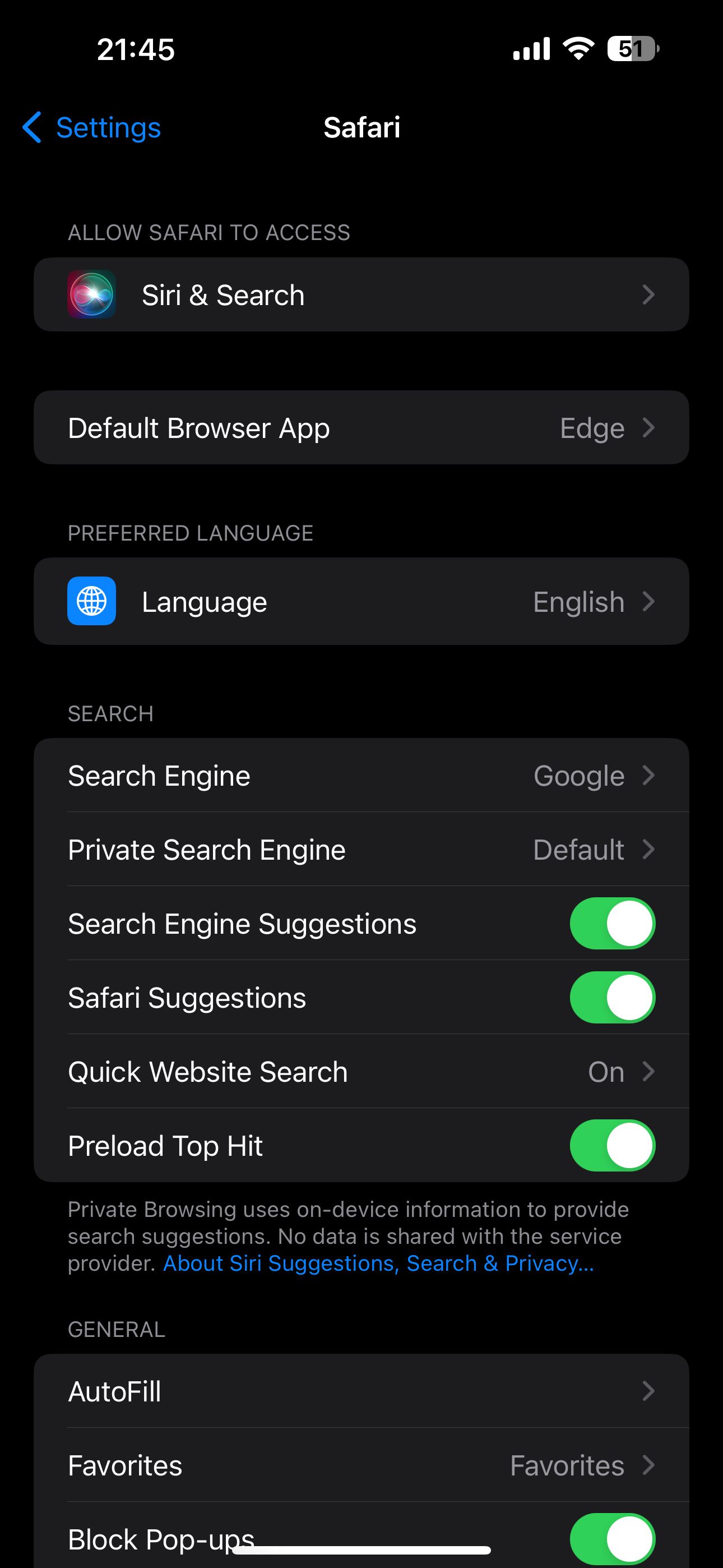The image depicts the settings menu of an Apple iPhone, primarily showcasing the configuration options for the Safari browser. The background of the menu is entirely black, with each selection section appearing in gray. 

At the top left corner, "21:45" is displayed, indicating the current time. The status bar shows four signal bars and a Wi-Fi icon, with the battery at 51%. 

The title "Settings" is highlighted in blue with a back arrow on the left side, followed by "Safari". The section title "Allow Safari to Access" introduces several options:
- "Siri & Search"
- "Default Browser App" set to "Edge"
- "Preferred Language," showing "Language: English"

Within the "Search" section:
- "Search Engine" is set to "Google".
- "Private Search Engine Default" is mentioned below.
- There is a toggle button for "Search Engine Suggestions," which is turned on (green).
- A similarly toggled-on button for "Safari Suggestions".
- "Quick Website Search" is set to "On", accompanied by an arrow.
- "Preload Top Hit" has an active toggle button.

In black text with gray letters, there is a message: "Private browsing uses on-device information to provide search suggestions. No data is shared with the service provider." A blue text link follows, reading "About Siri Suggestions, Search, and Privacy."

The "General" section includes:
- "Auto-fill"
- "Favorites"
- "Block Pop-ups," which is also toggled on.